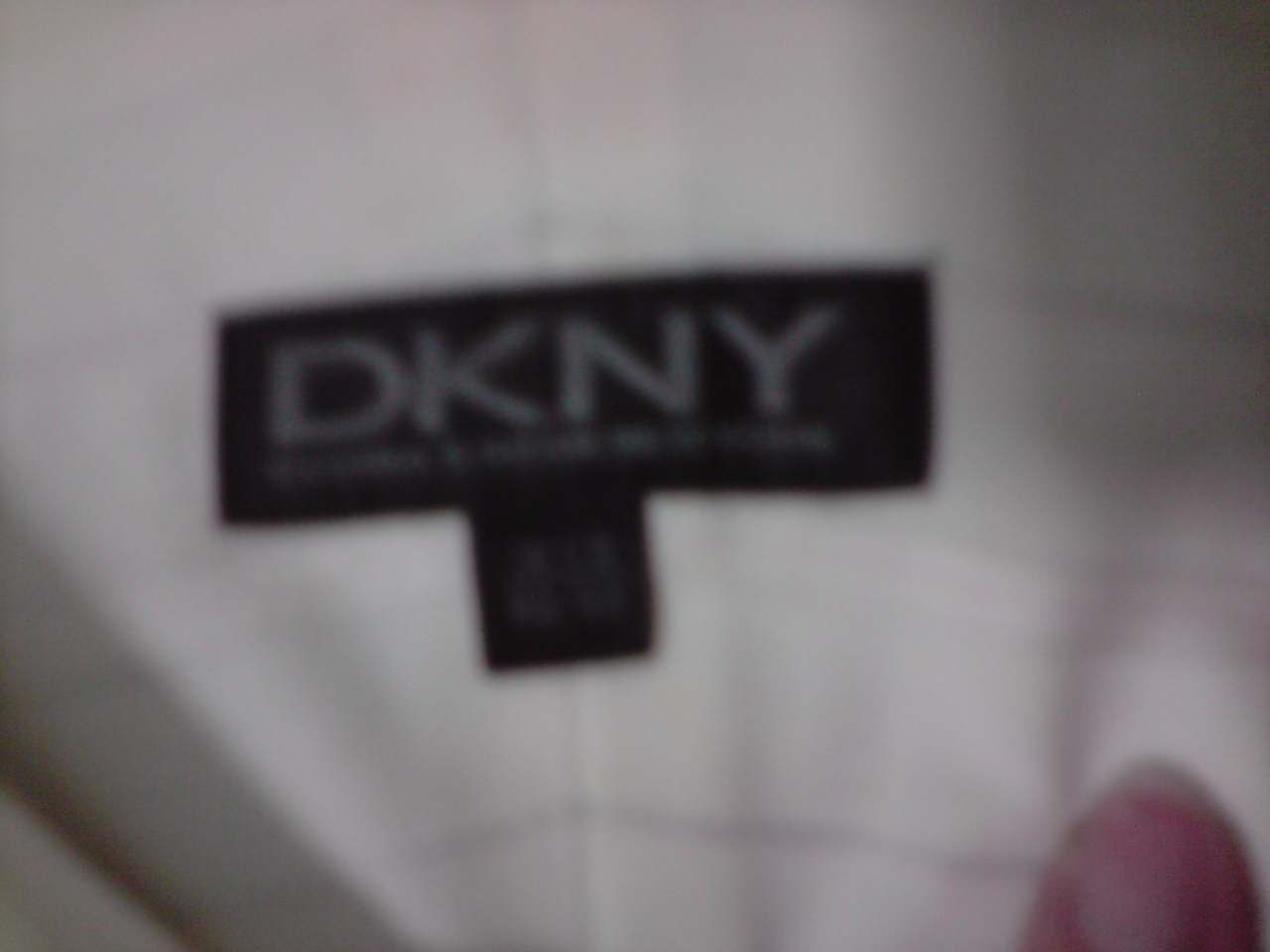The image is a color photograph that is very blurry and dark, making it difficult to discern clear details. Central to the image is a black, oblong label affixed to a surface that could likely be a garment, such as a shirt, which seems to have a gray and white windowpane design. The label prominently displays "DKNY" in white or gray capital letters. Below it, there is another smaller black rectangle with indistinguishable writing. The setting appears to be near a ceiling, indicated by the visible sections or lines of light panels on a white ceiling. In the lower right corner of the image, there is a partially visible oval shape that is hard to identify, and right beside it is what seems to be the tip of someone's thumb, likely a woman's, with a long nail casting a shadow. Additional shadows are present in the top right and bottom left corners of the picture, further obscuring the details and adding to the overall blurry effect.